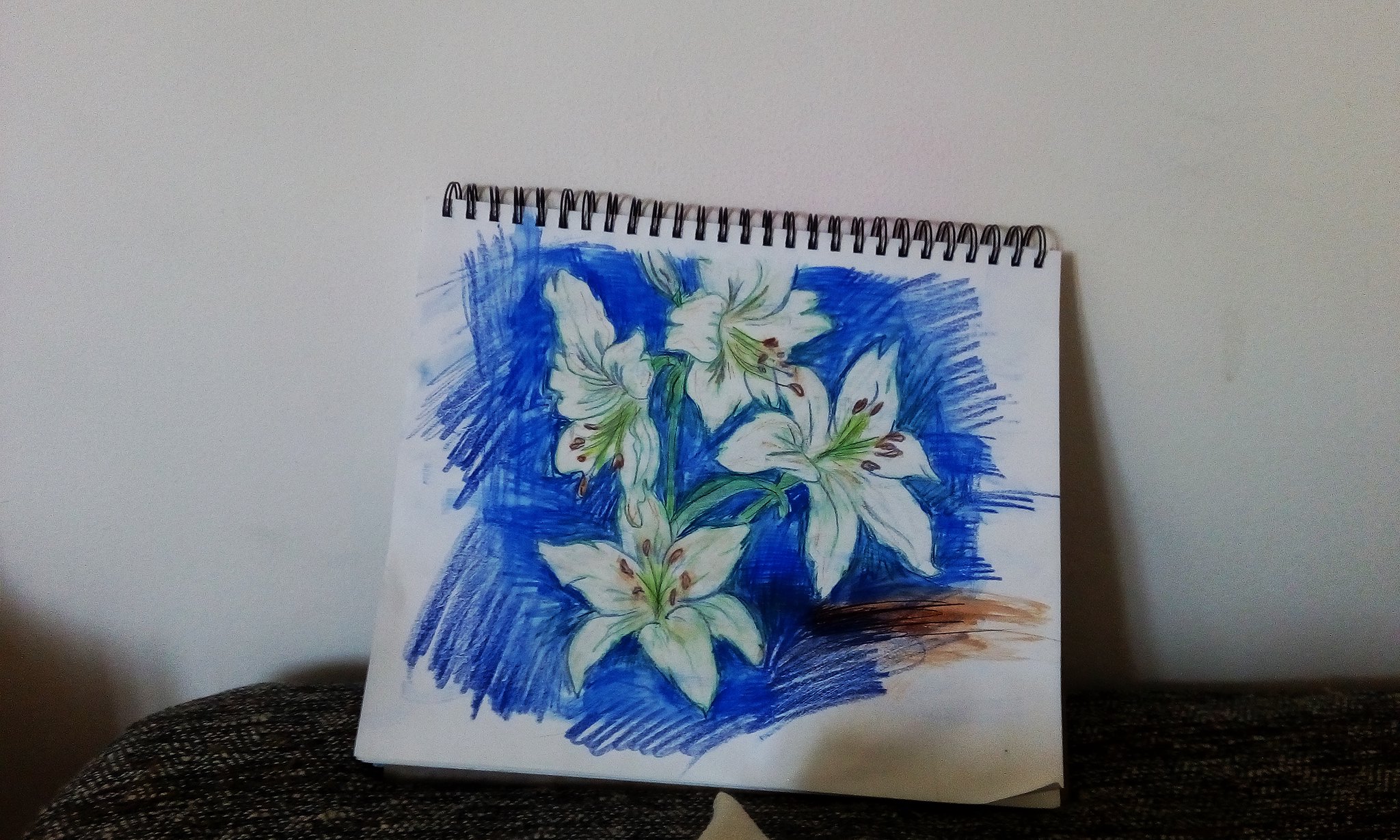A detailed indoor photo captures a sketchbook leaned against a white wall, propped up on dark gray or brown upholstered furniture. The sketchbook, which features coiled plastic rings on its left side, appears slightly open, showing the metal binding at the top. The artwork inside showcases a meticulously detailed drawing of four white lilies arranged in a square pattern, each facing different directions. These flowers are intricately accented with green shading at their centers and detailed with delicate petals and green stems. The blue background, evenly shaded with blue lines in various directions, contrasts with a subtle shading of brown on the right side of the sketch.